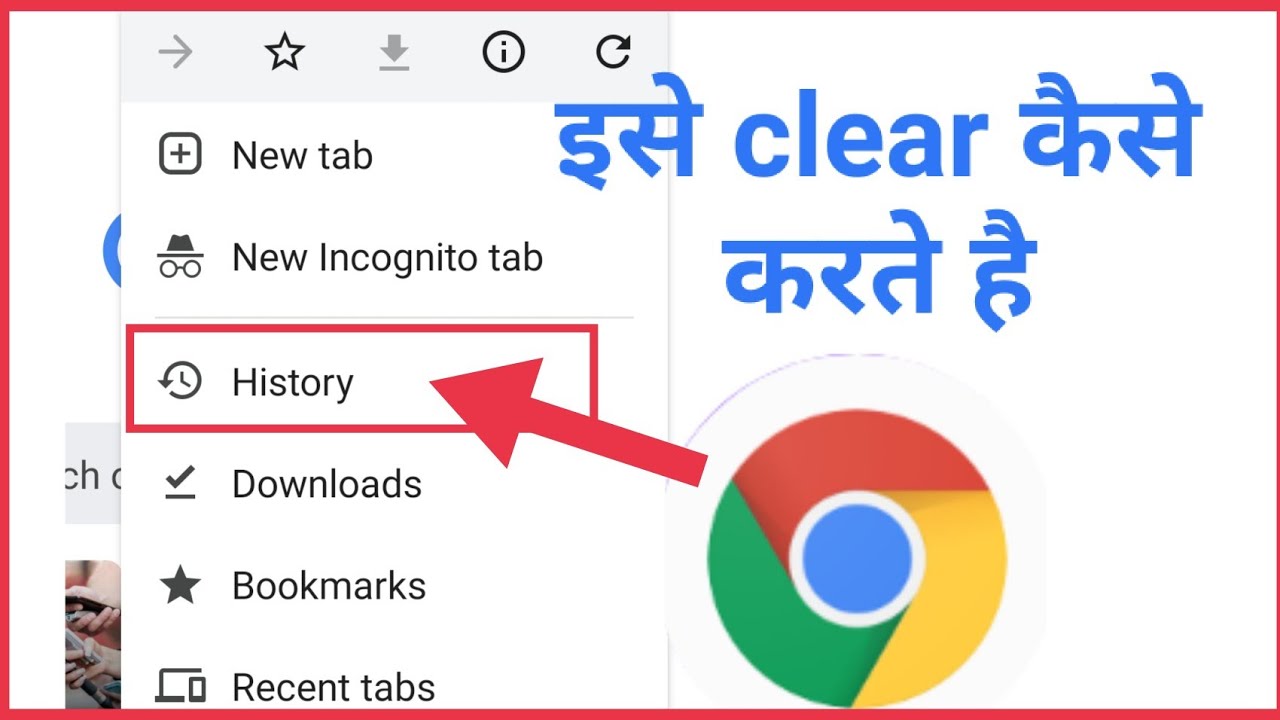A detailed caption for the given image could be:

"The image showcases a medium-red rectangular border framing a zoomed-in view of a Google Chrome interface, which is primarily intended to highlight the browser’s drop-down menu. The aspect ratio of the image is approximately 2:1. At the top of the browser window, there is a horizontal gray bar that spans about half the width of the image. This bar includes a series of icons: a forward gray arrow, a star, a downward gray arrow underlined in gray, a black user icon encircled in gray, and a refresh symbol that is nearly circular.

Beneath this bar, within the white menu area delineated by two vertical gray bars, several options are listed, including: 'New Tab,' 'New Incognito Tab,' 'History,' 'Downloads,' 'Bookmarks,' and 'Recent Tabs.' The 'History' option is enclosed within a red box, which has a red arrow pointing to it from the right side. In the same box, there is a Google Chrome logo, suggesting that this is an active menu item related to the browser’s history. The menu also contains some Asian characters next to the word 'Clear,' which is written in blue, indicating perhaps an option to clear browsing history or data."